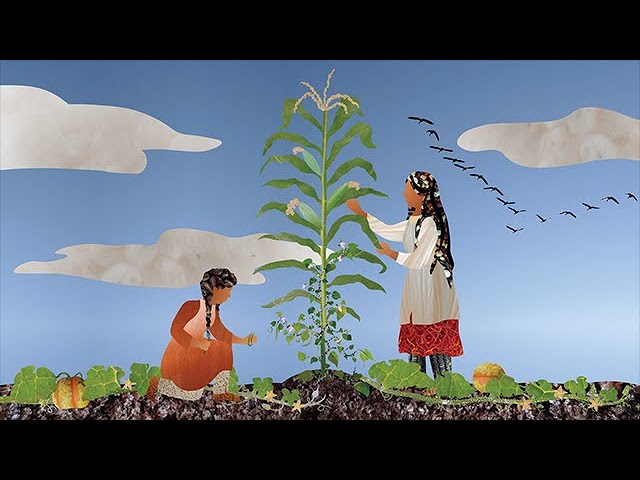This image is a vibrant, 2D artistic piece that intricately blends the qualities of painting and fabric artwork, resembling a mosaic or a pieced-together quilt. The focus is on a serene outdoor scene featuring two Native American women, adorned in old-fashioned red, white, and elaborately patterned robes. They are tending to a garden, embodying the age-old agricultural practice known as the "Three Sisters," where corn, beans, and squash thrive together. The woman on the right stands upright, attending to a large ear of corn, while the woman on the left kneels, caring for the nearby squash and beans that grow intertwined with the corn stalks.

Above, a clear blue sky adorned with soft, white clouds serves as the backdrop, accentuating the colorful garden below. Adding a dynamic touch, a V formation of black birds, likely geese, graces the upper right corner, enhancing the naturalistic tranquility of the scene. The artwork is rich with vibrant hues of blue, green, orange, yellow, and white, meticulously assembled to create a lively and harmonious depiction of traditional Native American life and agricultural wisdom.